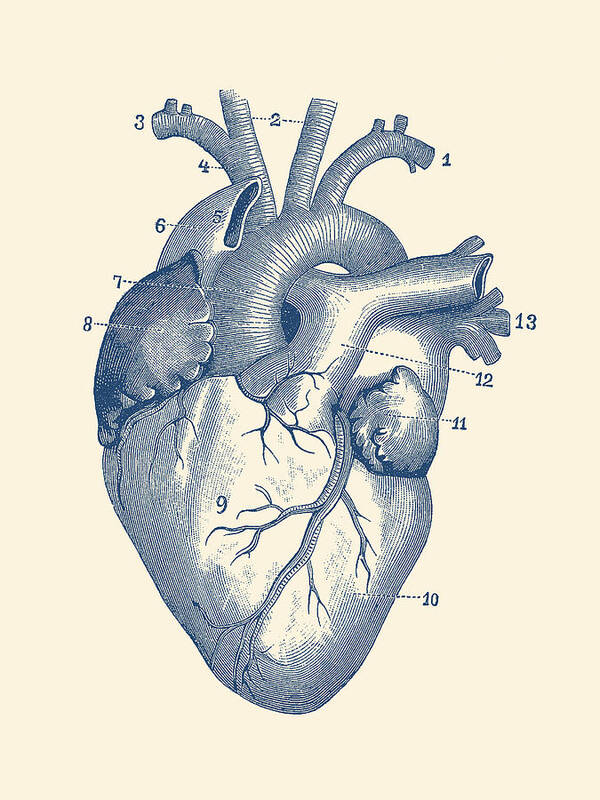This image is a detailed, hand-drawn illustration of the human heart, depicted in a bluish-gray hue on a creamy yellowish background. The drawing meticulously outlines the heart's shape, including its valves, arteries, chambers, and ventricles. Each part of the heart is numbered from 1 to 13, with dotted lines connecting the numbers to the specific sections they identify. While this particular image does not provide the names or descriptions of the numbered parts, it suggests that these are likely found on a separate page or accompanying legend. The background is a very pale pink, enhancing the focus on the heart's intricate details. The overall illustration serves as an informative visual representation, ideal for educational purposes.